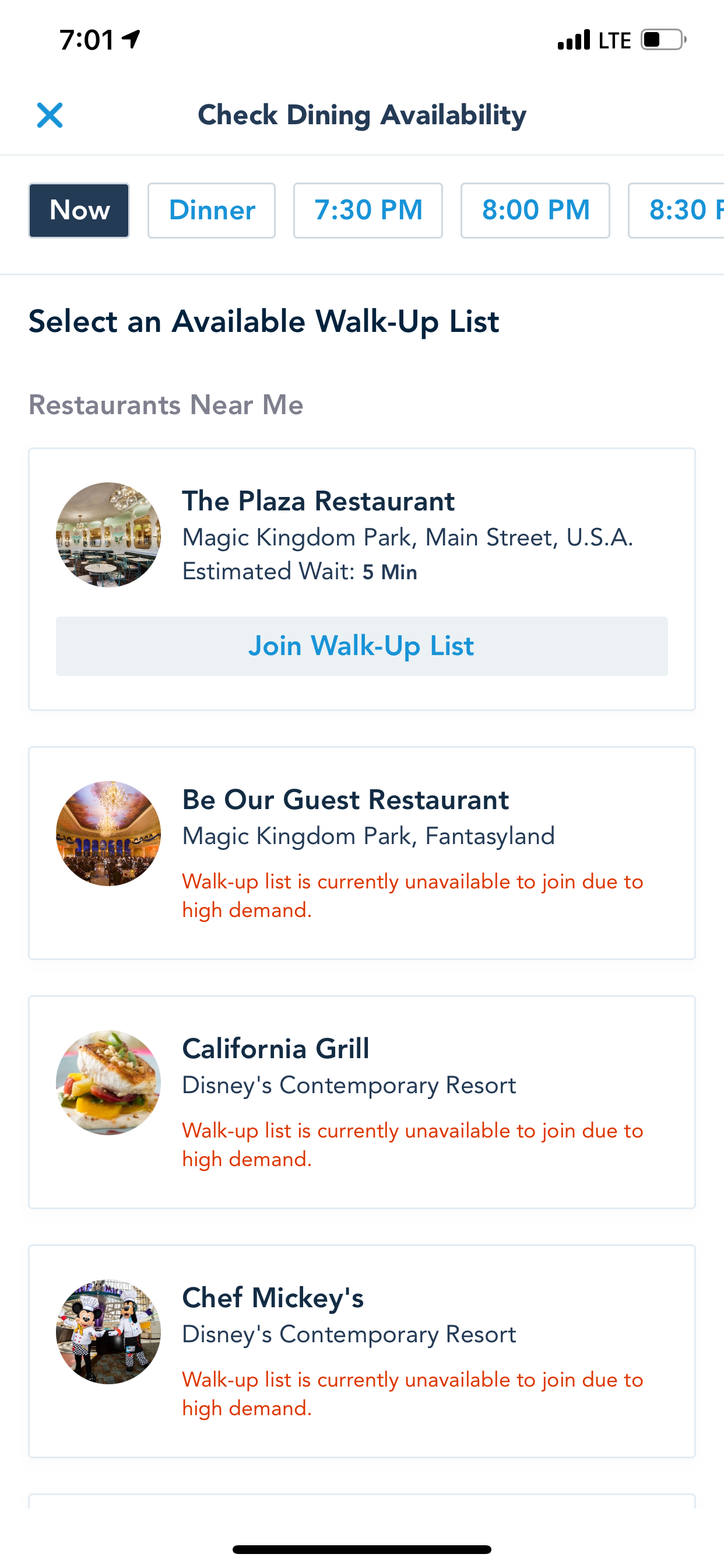The image displays a detailed interface for checking dining reservations and availability at various Disney restaurants. At the top, there is a timestamp indicating the current time as 7:01. Below it, there are options to check dining times and availability, with a highlighted box showing "Now." 

Following this, there are specific dinner time slots listed: 7:30 p.m., 8:30 p.m., and 8:00 p.m. Under these options, users can select from available walk-up lists, which include nearby restaurants, though there is a box with an unclear image.

Next, the image details restaurant options:
1. The Plaza Restaurant located at Magic Kingdom Park, Main Street USA, has an estimated wait time of five minutes. There is a button available labeled "Join Walk-Up List."
2. Be Our Guest Restaurant at Magic Kingdom Park, Fantasyland, states that the walk-up list is currently unavailable to join due to high demand.
3. California Grill at Disney's Contemporary Resort also notes that its walk-up list is unavailable to join due to high demand.
4. At the bottom, Chef Mickey's at Disney's Contemporary Resort similarly indicates that its walk-up list is currently unavailable to join due to high demand.